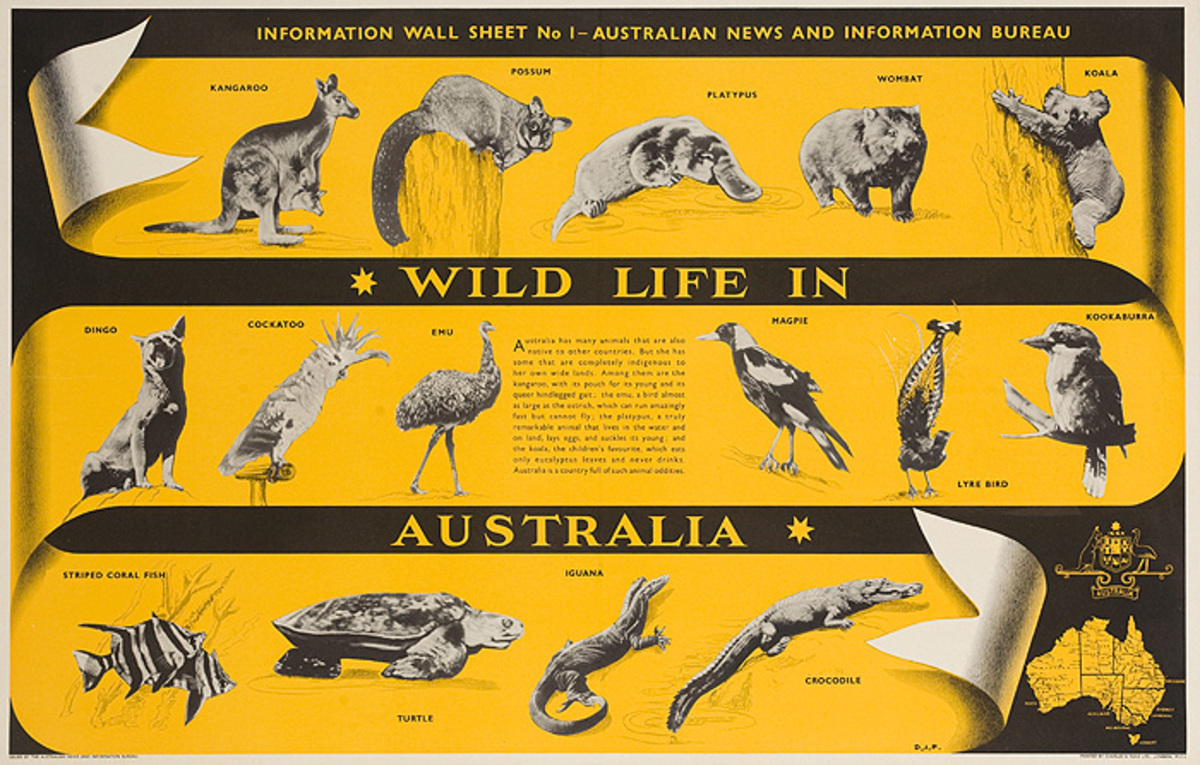This vintage-style educational poster, titled "Wildlife in Australia," features a compelling black background accentuated by three horizontal, scroll-like yellow ribbons. At the pinnacle of the poster, it states "Information Wall Sheet, Number 1, Australian News and Information Bureau." The poster showcases grayscale illustrations of diverse Australian wildlife arranged in three distinct rows, each labeled with species names in yellow font. 

In the first row, from left to right, you find a kangaroo, bushy-tailed possum, platypus, wombat, and koala. The second row includes a dingo, cockatoo, emu, magpie, lyrebird, and kookaburra. The third row presents a striped coral fish, turtle, iguana, and crocodile. A paragraph positioned in the second column provides an in-depth description of Australia's wildlife, elucidating the poster's educational intent.

In the bottom right corner, there's a mini map of Australia accompanied by an emblem that appears to represent the Australian Wildlife Association. This visually striking poster, dominated by its yellow and black color scheme, beautifully merges informative text with artistic illustrations, effectively capturing the essence of Australia's diverse fauna.